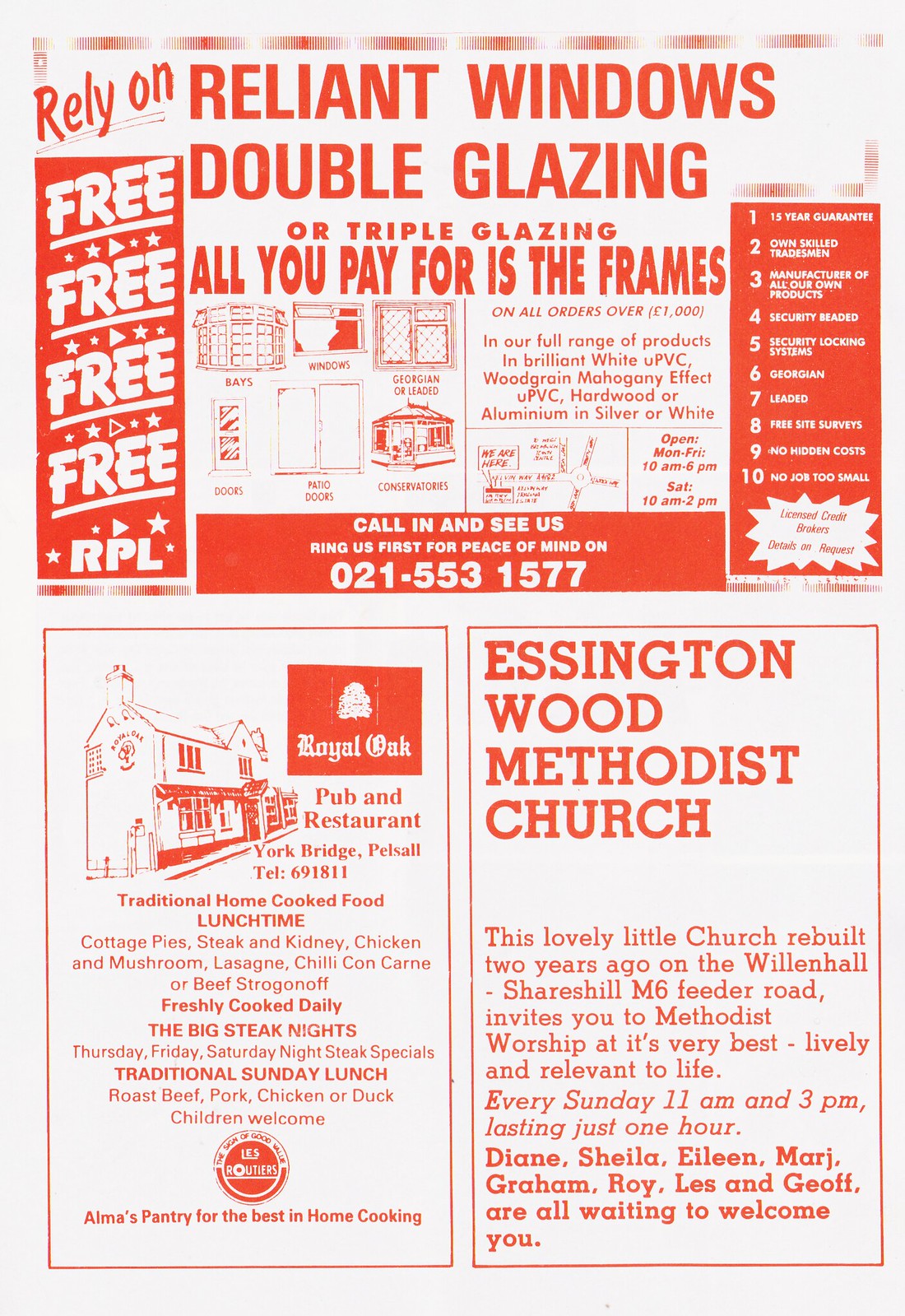This image depicts a page from a local paper featuring three vibrant advertisements, all in a striking orangish-red font against a white background. At the top, the prominent ad for Reliant Windows promotes double and triple glazing, stating, "All you pay for is the frames," accompanied by various images and detailed information about their window and frame services. On the bottom left, another ad highlights the Royal Oak Pub and Restaurant, providing its address, hours of operation, and special promotion nights, aiming to attract food enthusiasts. On the bottom right, an ad for Essington Wood Methodist Church describes the church's location along Woollen Hall, Shares Hill, near the M6 Feeder Road. It details the inviting nature of their worship services every Sunday at 11 am and 3 pm, emphasizing a lively and relevant experience. The page is filled with comprehensive text, making it visually informative and engaging.